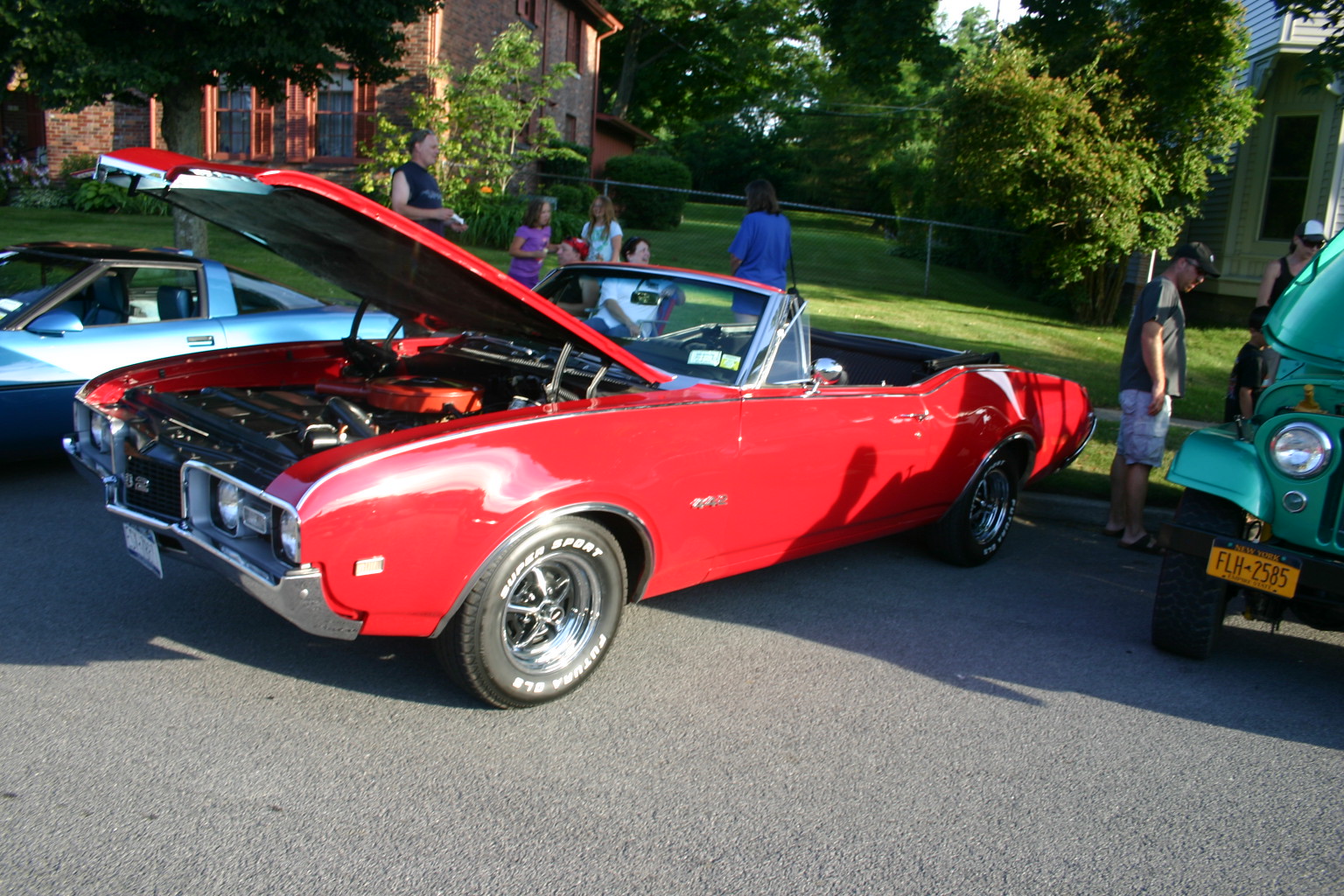The image depicts a vibrant outdoor setting, likely from a classic car show, with a striking red vintage convertible as the focal point. The car, reminiscent of models from the late 70s to early 80s, has its hood popped open, revealing its intricate engine along with the roof retracted, accentuating its classic design. The car’s elongated body and spacious interior create a striking and nostalgic presence. 

Surrounding the red convertible, a diverse crowd of adults and children engage in lively conversations and leisurely strolls, adding to the communal atmosphere of the sunny day. Adjacent to the convertible, on the left, is a partially visible blue Corvette, while on the right, stands what appears to be an older green Jeep, beside which a man dressed in a grey top, light blue shorts, and sliders is seen examining the vehicles.

The background features lush greenery with a large grassy area and several tall trees providing shade. You can spot a few people walking towards this verdant expanse. In front of the parking lot, a brown building is partially visible alongside what seem to be houses, partially obscured by bushes and a chain-link fence, contributing to the neighborhood-like ambiance. The image captures a dynamic blend of classic automotive charm and a vibrant community gathering.